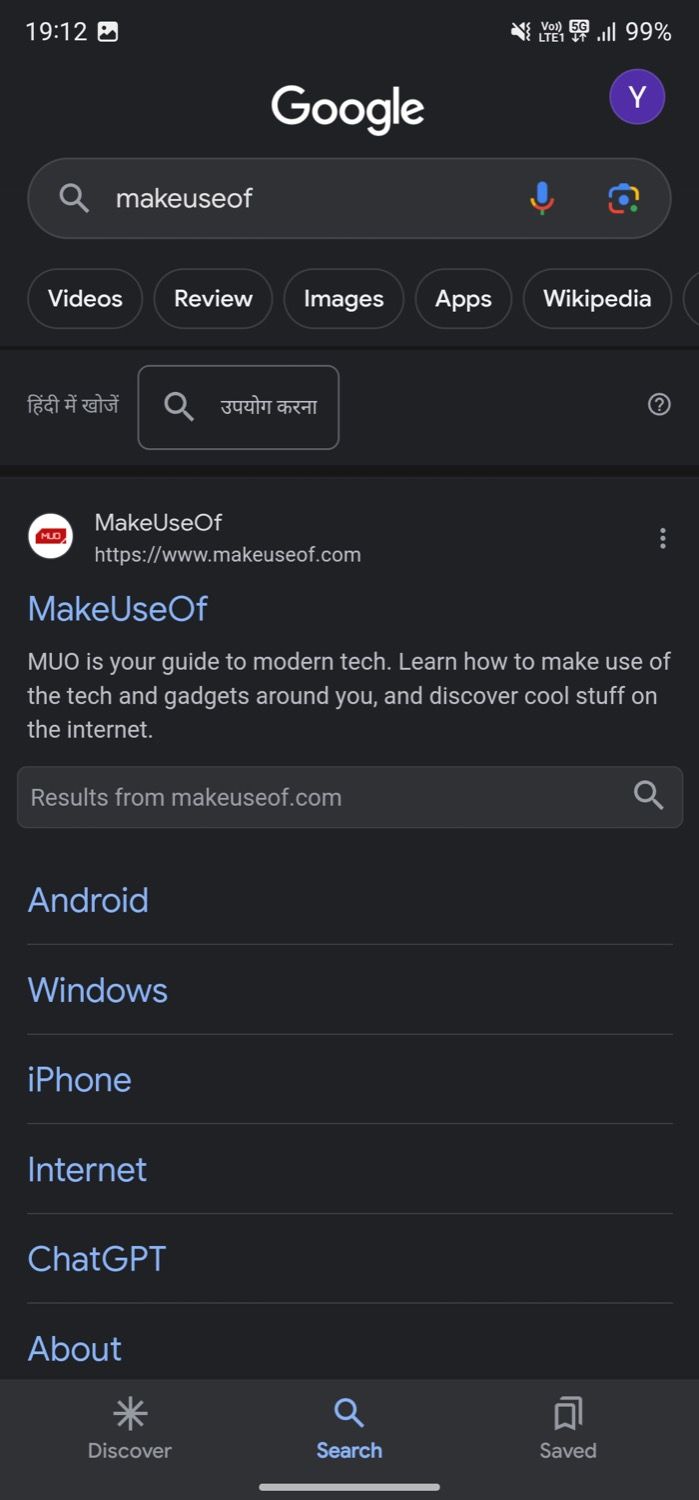A user has conducted a Google search for the term "makeuseof" as a single concatenated word on a smartphone. The device is set on a light-themed background, and the screen displays the interface of the Google search results page. The time shown at the upper left corner of the screen is 19:12, accompanied by a small photo icon. At the upper right corner, indicators include a volume icon (muted), LTE connection, a 5G logo, 4 signal bars, and a battery level at 99%. Adjacent to these icons is a purple circular user icon with the letter "Y", indicating the logged-in Google user.

The central part of the screen features the Google search field with an added microphone icon for voice searches. An image search icon is also present nearby. Below the search bar, various browsing options like "All," "Images," "Videos," "Reviews," "Apps," and "Wikipedia" are listed, enabling different forms of content exploration.

The primary search result is from the website "makeuseof.com" with a brief description: "MakeUseOf (MUO) is your guide to modern tech. Learn how to make use of the tech and gadgets around you and discover cool stuff on the Internet." The displayed search results include links to various sections of the website covering topics related to Android, Windows, iPhone, internet, ChatGPT, and other technology areas.

At the bottom of the screen, standard navigation options "Discover," "Search," and "Saved" are visible, providing convenient access to different parts of the Google app. A portion of the screen also contains text in an unknown language, potentially Hindi or another Indian dialect, but it remains unreadable to the user.

This detailed caption incorporated all visible elements into a coherent description, presenting a clear picture of the device’s screen and the search circumstances.